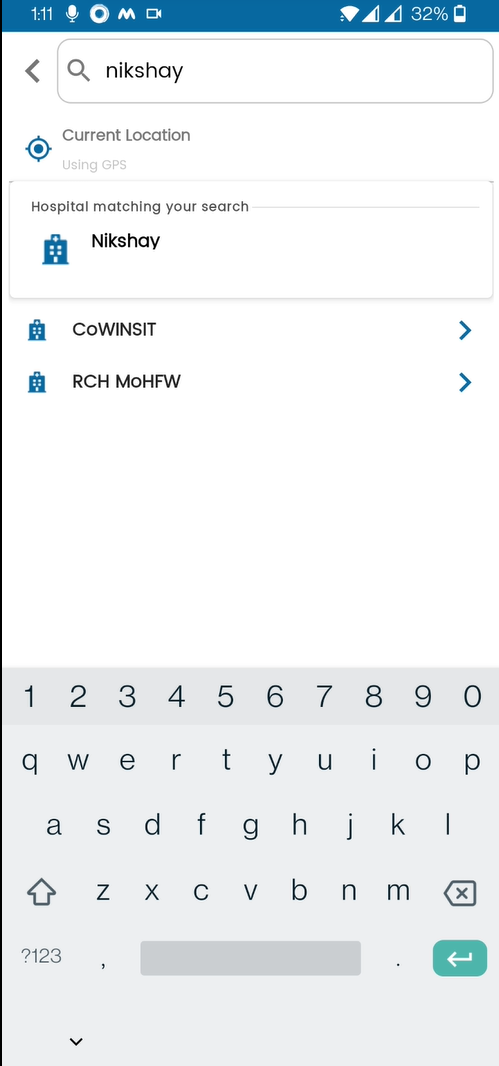This screenshot, captured from an Android smartphone, features an interface likely related to healthcare or hospital services. At the top, the status bar displays the time as 1:11, with no indication of whether it's a.m. or p.m. To the left, there are symbols for an active microphone and camera, suggesting both are in use or available. An 'M' icon might represent the app being used, followed by another camera icon, potentially indicating that recording is taking place or that the camera is active.

To the far right, the status bar shows a full Wi-Fi signal, indicating a strong wireless connection. Next to it are two data signal bars, each representing a SIM card configuration. The first SIM card signal is approximately at 75% strength, while the second is at about 50%. Battery life is clearly indicated at 32%, with the corresponding battery icon showing about one-third remaining charge.

The app or website displayed in the screenshot appears to focus on connecting users with various hospitals at a specific location, suggesting functionalities related to matching or finding healthcare facilities.